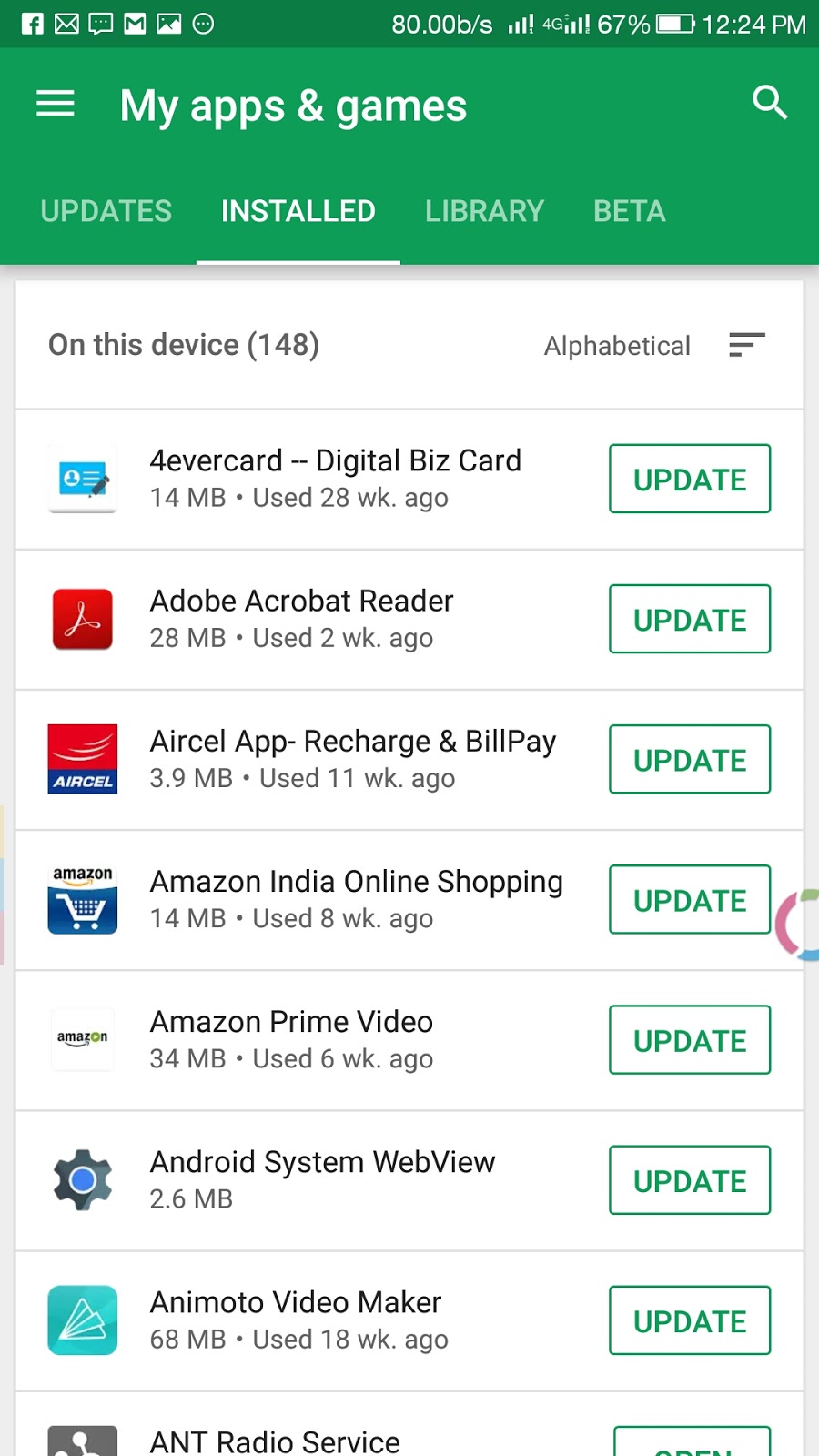Screenshot of a phone displaying the "My Apps & Games" panel. The interface is mostly dark with a medium dark green line at the top and a lighter green area where the title is located. 

At the top of the screen, there are icons for Facebook, an envelope, a speech bubble, and Gmail, along with an image viewer, three dots in a circle, and a status display showing "80.00 B/s". Signal strength is shown with four bars next to a "4G" indicator, followed by another set of four bars and a battery icon indicating 67% at 12:24 PM. 

A hamburger menu labeled "My Apps & Games" is on the left with a magnifying glass on the right. Below this, the menu options "Updates," "Installed," "Library," and "Beta" are displayed, with "Installed" being selected, indicated by a white bar.

The list of installed apps includes a total of 148 items, shown alphabetically. Each app is listed with its icon on the left, followed by its name, size, and last usage. On the right side of each entry, there are three staggered bars for more options. Beside this, a green-outlined "Update" button with white capital text is visible for some apps. The visible apps in the list include:

1. Forever Card Digital Biz Card - 14 MB, last used 28 weeks ago
2. Adobe Acrobat Reader
3. Aircel App Recharge and Bill Pay
4. Amazon India Online Shopping
5. Amazon Prime Video
6. Android System Web Viewer
7. Moto Video Maker
8. Anti Radio Service